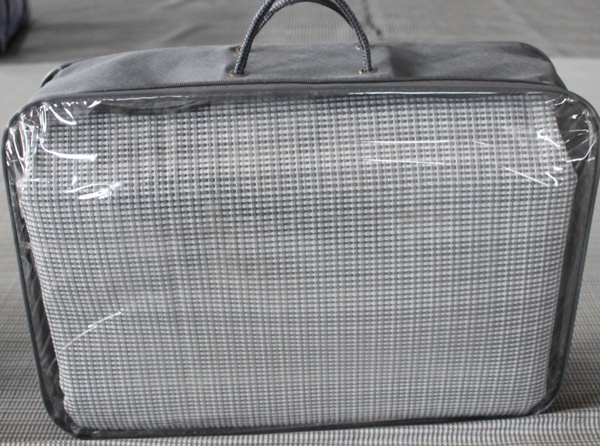The photograph captures a product encased in a bag with soft grey fabric sides and a transparent plastic front panel, allowing a clear view of its contents. The bag, oriented upright with two grey rope handles threaded through grommets at the top, rests on a fabric surface that closely matches the light and dark grey woven material inside the bag. This textured material, possibly a cloth, rug, or bedspread, is flexible and mirrors the fabric pattern of the ground beneath the bag. The background is dimly lit and features some wrinkles in the fabric, along with other indistinct objects. The image, taken in black and white, accentuates the shiny highlights on the plastic front, emphasizing the transparent panel aimed directly at the camera. The entire scene is devoid of text or labels, adding a sense of ambiguity to the exact nature of the bag's contents.